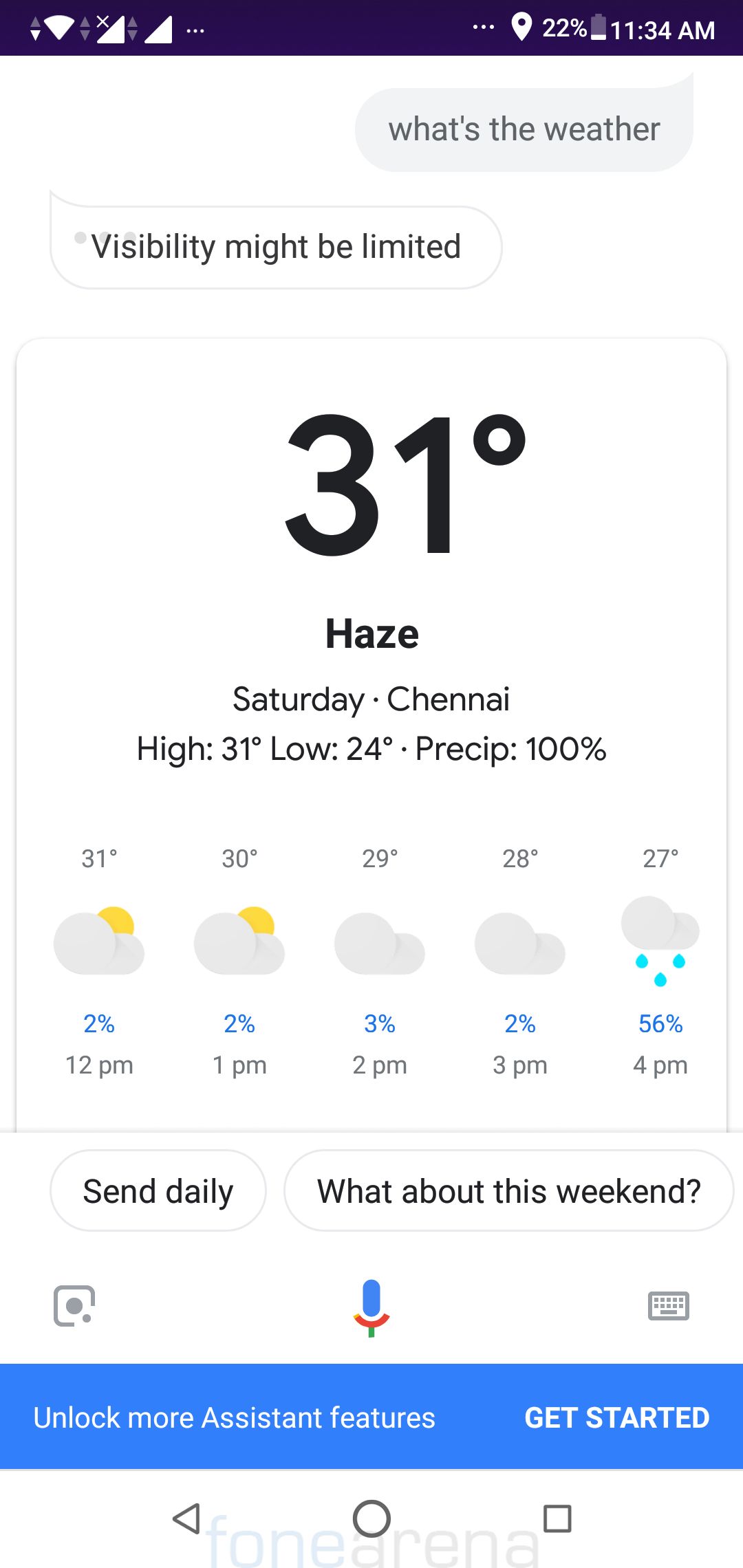This image, taken on a smartphone, prominently displays a snapshot of a weather application at 11:34 a.m. Various phone icons are visible at the top of the screen, confirming the mobile device. 

In the chat interface, a user initially inquires, "What's the weather?" This text appears in gray, indicating it was typed by the user. The response, in white text, states, "Visibility might be limited." 

A gray-outlined box provides comprehensive weather details: 

- The current temperature is 31°C.
- Haze is prevalent.
- The location is Chennai.
- It's Saturday.

Additional weather stats include:

- High of 31°C
- Low of 24°C
- 100% precipitation

The screen then transitions into an hour-by-hour forecast:
 
- At 12 p.m., it is 31°C with a 2% chance of precipitation, and the weather is partly sunny.
- At 1 p.m., it is 30°C with a 2% chance of precipitation, and the weather remains partly sunny.
- At 2 p.m., it is 29°C with a 3% chance of precipitation, under cloudy skies.
- At 3 p.m., the temperature drops to 28°C with a 2% chance of precipitation, and continues to be cloudy.
- By 4 p.m., it is 27°C with a significant 56% chance of precipitation, signifying rain.

At the bottom of the interface are two interactive buttons: "Send Daily" for daily updates and "What about this weekend?" for weekend weather details. Below these, a long blue box features a microphone icon with a prompt to "Unlock for more Assistant features" alongside a "Get Started" button.